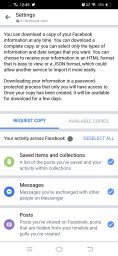The image captures a smartphone screen displaying a Facebook settings section. At the very top, a black bar showcases indicators such as the current time, Wi-Fi signal strength, and battery percentage. Below this bar, the screen is divided into two main sections, with various settings options and instructions for downloading data in different formats like HTML and JSON.

Prominently, there is a grey back arrow that allows users to navigate to the previous screen. Within the settings context, one section is highlighted in blue and labeled "Request Copy," suggesting a feature to request a copy of personal data. Nearby, the text "Your Security Across Facebook" is visible, indicating a focus on user security options.

Alongside these elements, there are various icons representing different categories: a green icon for "Saved Collections," a blue icon for "Messages," and a purple icon for "Posts." These icons guide users to specific sections within the settings.

At the bottom of the screen, multiple buttons are set against a white background with black text: one features horizontal white lines, another is a simple circle, and the third is a backward-facing arrow. Additionally, there is a "Deselect All" button in blue, allowing users to quickly manage their selection options.